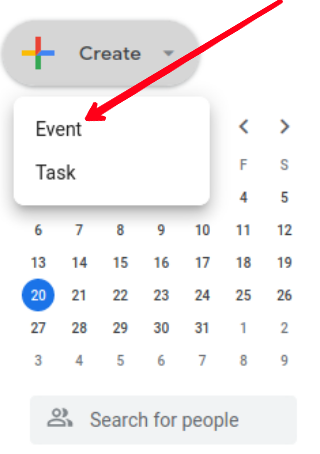This image captures a portion of a Google Calendar interface, featuring a white background typical of the platform. The calendar grid is displayed, with the dates denoted in a medium gray font. 

In the upper left corner, there is a gray rectangle with rounded corners that contains the word “Create” in its center. To the left of this rectangle, there is a plus sign composed of the Google signature colors: yellow, red, blue, and green.

Below this section, there is another rectangle with a white background and a light gray outline. At its top left, it displays the word “Event” followed by “Task” underneath it. A red arrow, originating from the upper right corner of the image, points directly to the word “Event.”

On the calendar itself, the date 20th is highlighted with a blue circle, and the number 20 is prominently displayed in white within the circle.

At the very bottom of the image, there is a search bar with a light gray background featuring the phrase “Search for people” in gray text. To the left of this text, there is an icon representing people, depicted as small circles atop schematic shoulder drawings.